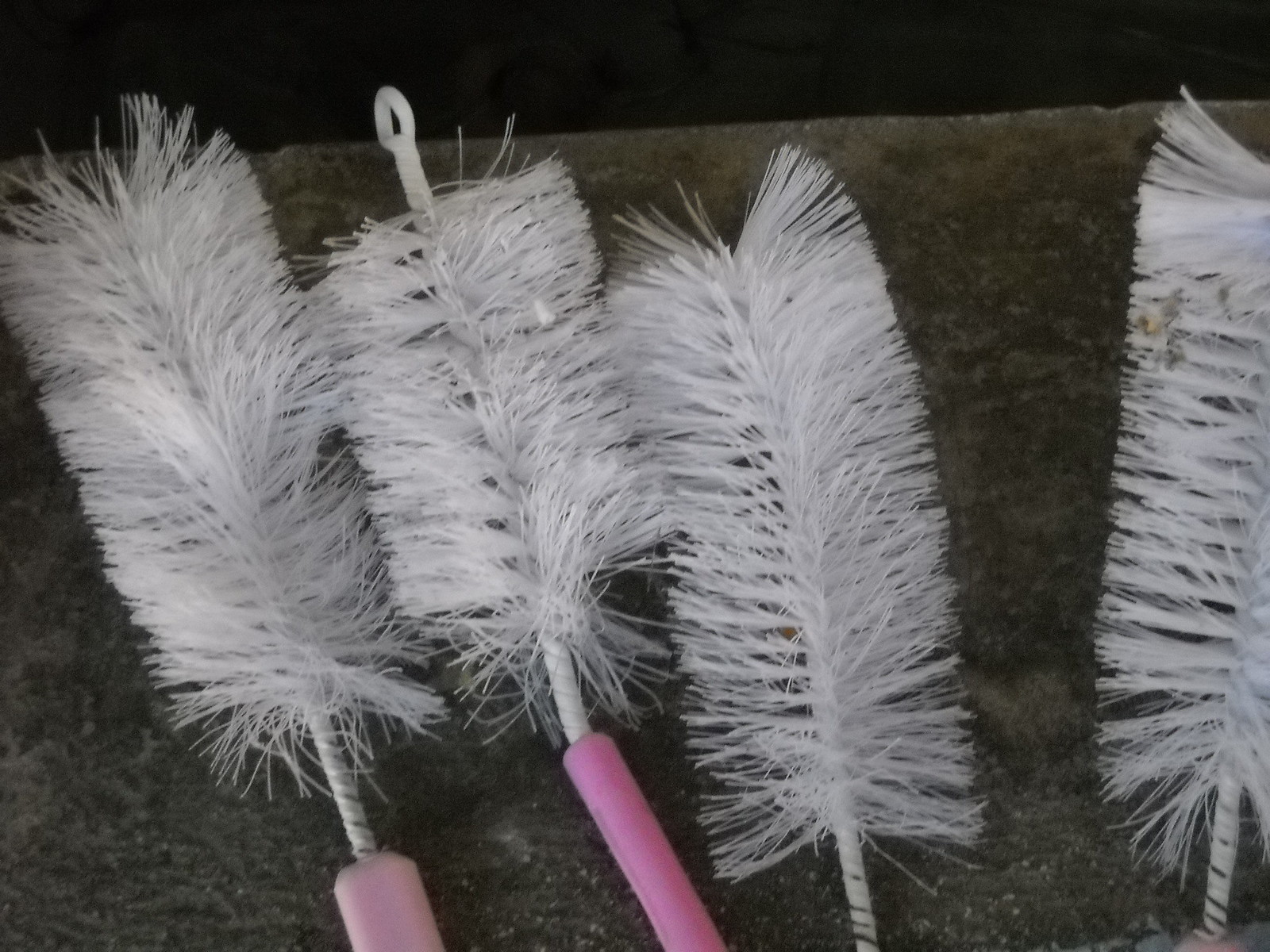The image features a close-up of four well-used bottle cleaning brushes, possibly for baby bottles, showcasing varying degrees of wear. All the brushes have white bristles that are frayed and scattered in different directions, indicating extensive use. The two brushes on the left have clearly visible handles—one in light pastel pink and the other in a more vibrant hot pink. The third brush on the right displays only a hint of its pink handle, while the handle of the fourth brush remains obscured. These brushes rest on a stone-like countertop, which appears to be a mixture of gray, black, and white hues. The background is dark, suggesting the edge of the countertop or an unlit area beyond.